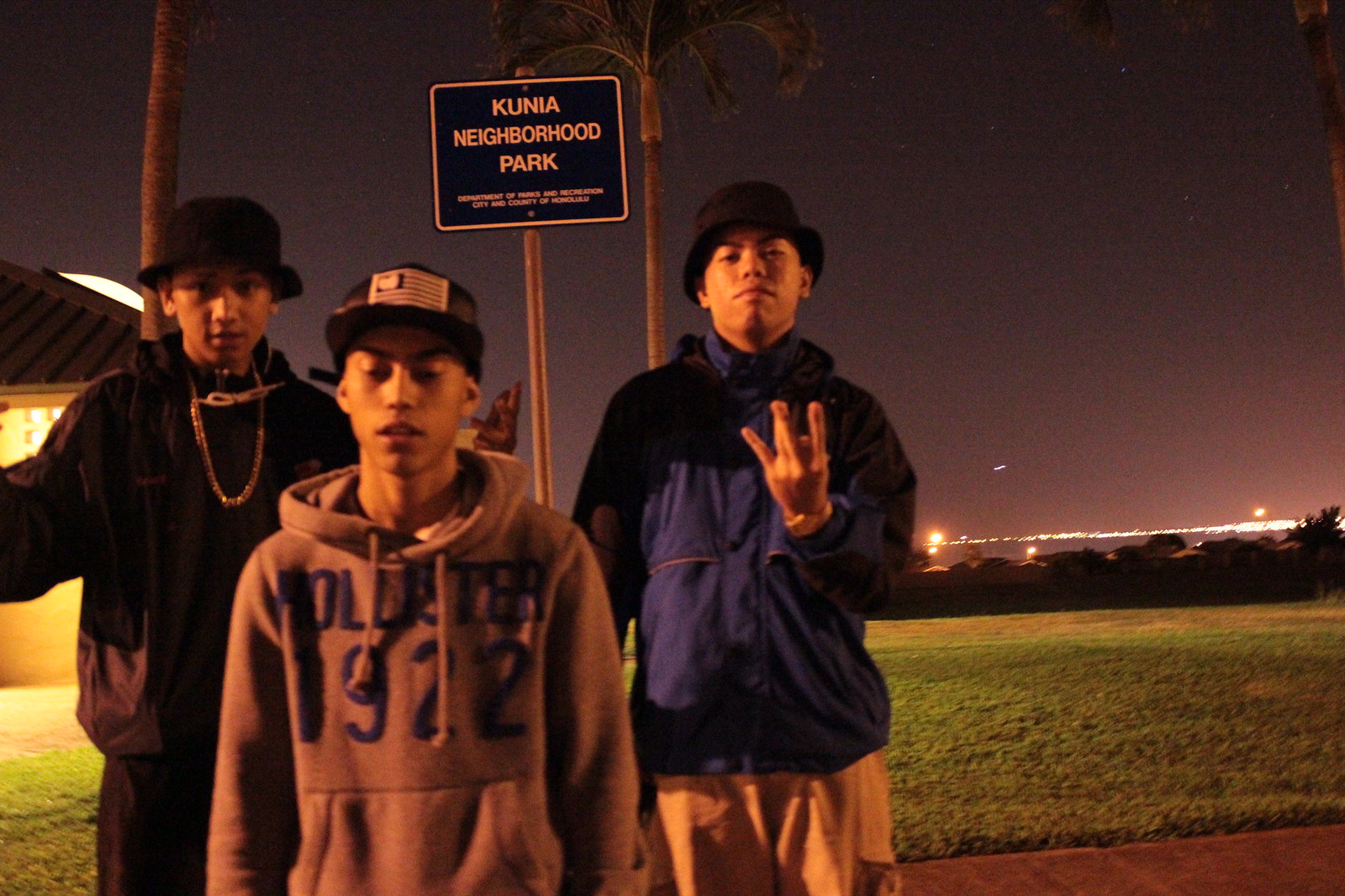This nighttime color photograph captures an urban outdoor scene with significant light pollution, casting a purplish haze over the sky and obscuring any stars. The scene is set near Coonagh Neighborhood Park, as indicated by a sign in the background. A few palm trees and a building with illuminated lights are also visible in the distance, along with streetlights that blend into the night.

In the foreground, standing on a pavement bordered by green grass, are three teenage boys, each wearing a different style of hat along with hoodies or jackets. The first boy on the left is dressed in a black sweatshirt, a gold necklace, and a black hat. The boy in the middle sports a brownish hoodie with the text "Volunteer 1972" and has his eyes closed, giving off a more serene vibe. Meanwhile, the third boy on the right wears a blue jacket, khaki shorts, and a hat, and appears more animated, holding up three fingers towards the camera. The atmosphere conveys a blend of urban landscape and youthful energy amidst the quiet of night.